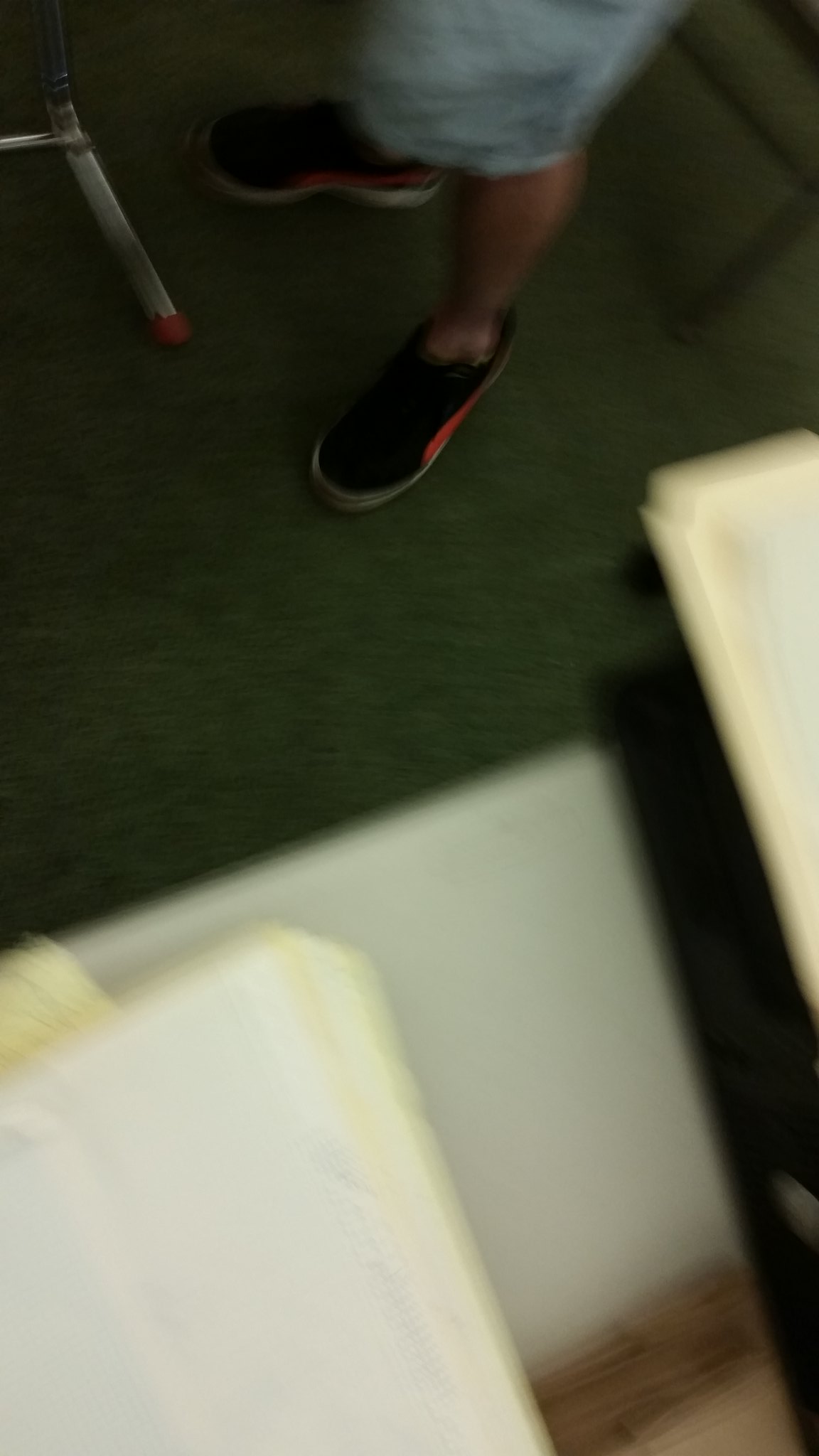This is a vertically-oriented, slightly blurry photograph likely taken with a phone held upright. In the upper left corner, there is the leg of what appears to be a desk chair, suggesting the setting is a classroom. Dominating the top third of the image are the feet and legs of a person standing behind the chair. This person is wearing black sneakers with a distinctive red stripe just above the white soles. They appear to be either not wearing socks or wearing very short ones. Their attire includes wide-legged denim shorts that end above the knee. The lower portion of the photograph is more indistinct, showing what looks like the top of a desk cluttered with papers. The flooring beneath the desk and the person is green carpet.